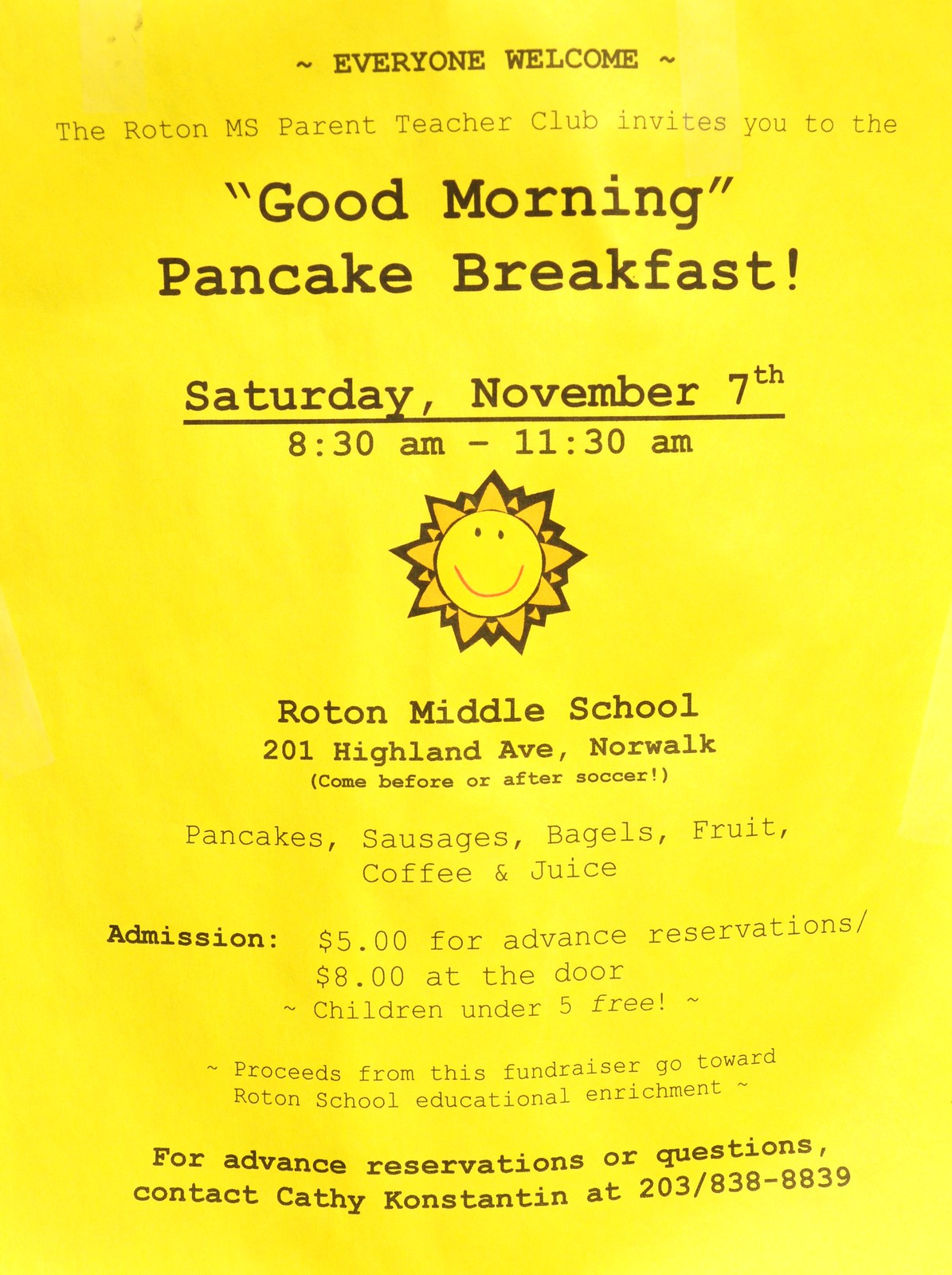The image is a detailed yellow flyer advertising the "Good Morning Pancake Breakfast" organized by the Roten Middle School Parent Teacher Club. The text, in black font, warmly invites everyone to the event scheduled for Saturday, November 7th, from 8:30 AM to 11:30 AM at Roten Middle School, located at 201 Highland Ave, Norwalk. A cheerful cartoon sun decorates the flyer, symbolizing a bright morning. Attendees are encouraged to visit either before or after their soccer activities. The delicious breakfast menu includes pancakes, sausages, bagels, fruit, coffee, and juice. Admission is set at $5 for advanced reservations and $8 at the door, with children under 5 admitted for free. Proceeds will benefit Roten Educational Enrichment. For advanced reservations or inquiries, you can contact Kathy Constantine at 203-838-8839.